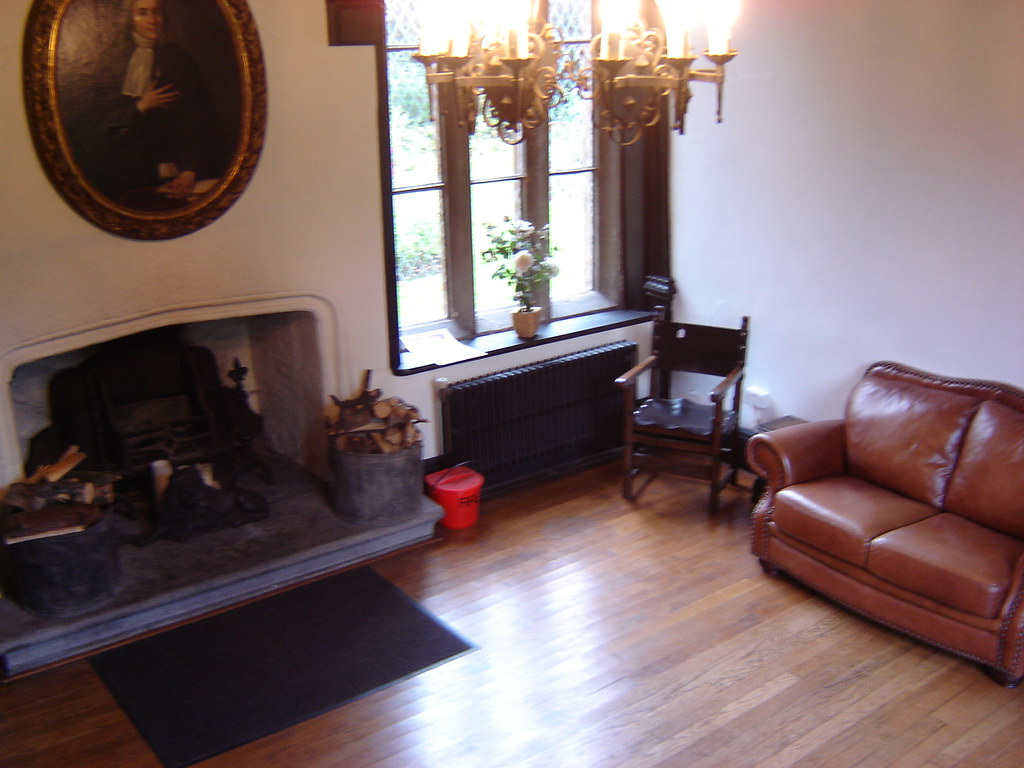The photograph captures a beautifully arranged, classical-looking living room characterized by a blend of Victorian design elements and modern touches. The center of the image showcases the corner of the room where a multi-pane glass window set in a black and gray frame allows sunlight to stream in, casting a warm glow on the shiny wooden floor. Below the window, a black radiator stands ready to provide warmth during colder months, while a windowsill above holds both fake and real flowers.

To the left side of the image, there's a white-painted wall adorned with an oval-shaped vintage painting of a figure in elaborate attire, lending a touch of historical charm. Beneath the painting, a fireplace stocked with logs and possibly a coal bucket sits ready for use, adding to the room's cozy ambiance. A tidy mat lies in front of the fireplace, accompanied by a bucket full of chopped firewood, hinting at a readiness for a crackling fire.

On the right side, against another white wall, sits a light brown, double-seated leather couch, exuding comfort. Next to it, in the corner, a black wood chair with a leather seat completes the seating arrangement. Above this setup, a bright chandelier hangs from the ceiling, illuminating the room with its warm, inviting light. The overall scene is of a clean, tidy, and inviting living room, with an aesthetic that beautifully merges Victorian elegance with contemporary cleanliness and warmth.